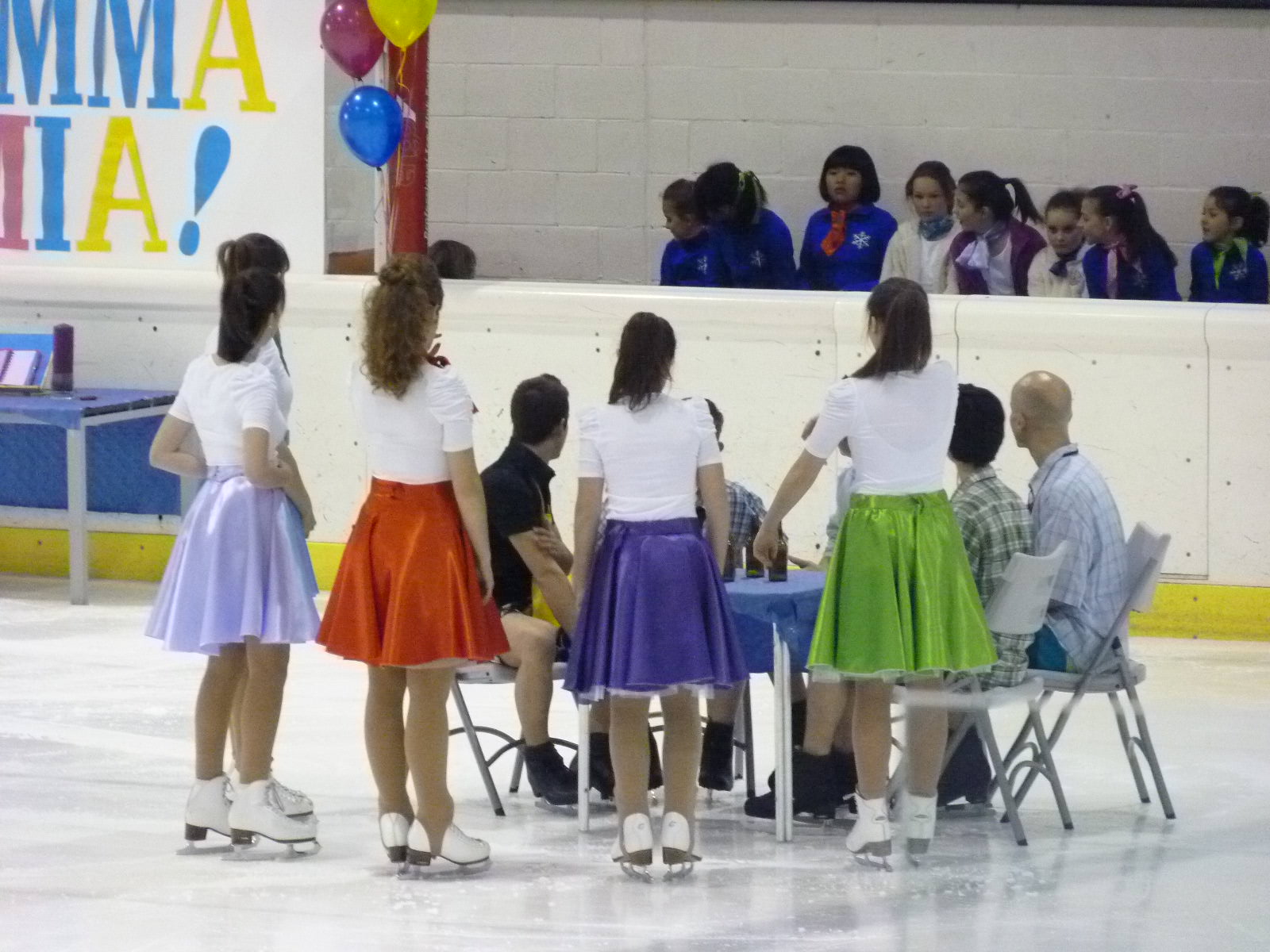In the image, a bustling scene unfolds set on what appears to be an ice rink. At the center of the rink stands a table adorned with a blue tablecloth, surrounded by several white fold-up chairs. Sitting in these chairs, you can see about five or six men dressed casually in flannel and polo shirts, all wearing black ice skates. Encircling the table are several women dressed in white quarter-sleeve shirts paired with colorful knee-length skirts in shades of light purple, red, dark purple, and green, each woman wearing white ice skates.

The women and men are gathered in what appears to be an earnest discussion, their backs faced towards something beyond the camera, situated behind the rink’s barrier. The rink’s background shows a white brick wall and the boundary of the ice rink itself, where a group of young girls watches attentively. These onlookers are donned in jacket uniforms—blue, white, and purple respectively—each observing the scene with interest.

To the left side of the image, part of a sign can be seen, displaying the letters "M-M-A" and "M-I-A," likely reading "Mamma Mia!" in colorful fonts of blue, yellow, and red. Accompanying the sign are matching blue, yellow, and reddish-purple balloons tethered by a string. Below this festive signage is another table draped in a blue tablecloth, upon which rests a cylindrical object and what appears to be a book, adding more intrigue to the scene.